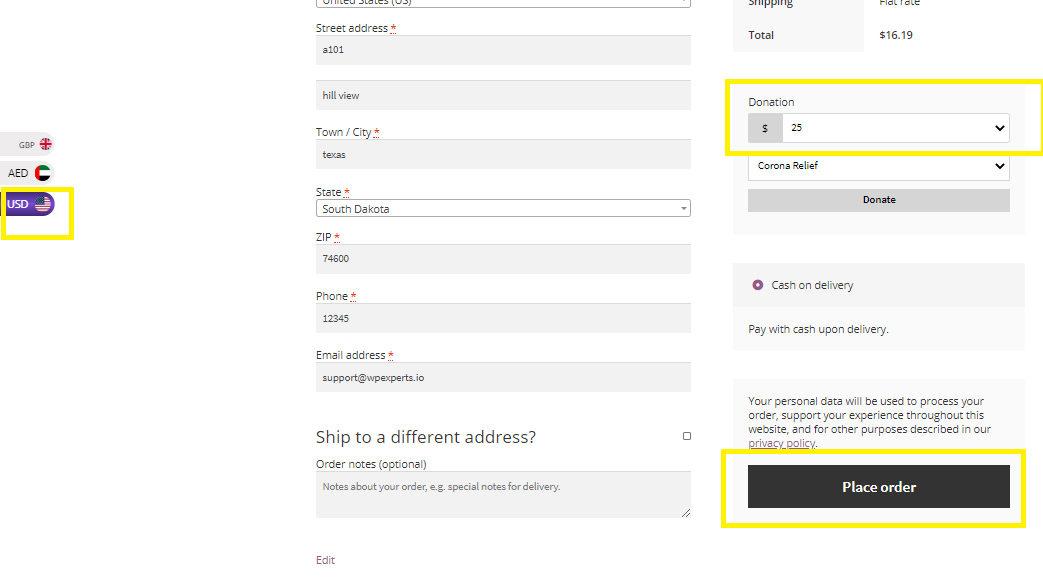This screenshot captures a website's order form menu, designed to collect customer information for placing an order. On the far left side of the interface are three currency selection tabs. The bottom tab, highlighted with a yellow square, is selected and displays the USD currency option, indicated by a blue background and white text, alongside an American flag. Above this are options for AED, marked with the respective flag, and GBP, paired with a British flag.

To the right of the currency options is an entry form for inputting address details. The form contains fields labeled "Street Address," where the sample entry is "A101 Hillview, Texas State, South Dakota, ZIP Code 74600." The "Phone Number" field is filled out with a placeholder “12345.” In the "Email Address" field, the sample text "support@webexperts.io" is provided. Additionally, there is a checkbox and field labeled "Ship to a different address," followed by an "Order Notes (Optional)" section. In this section, placeholder text reads "Notes about your order, e.g., special notes for delivery." The layout and specific details provided offer clarity on how to complete the form accurately.